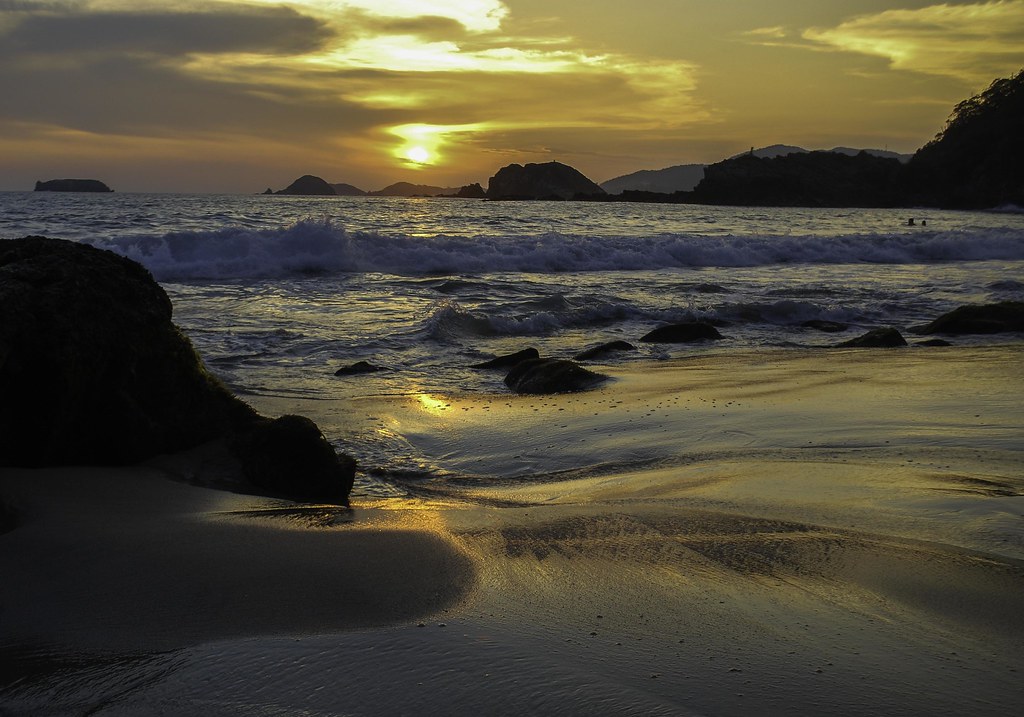An early morning sunrise (or potentially a late evening sunset) over a tranquil ocean takes center stage in this captivating image. The focal point is the vibrant blue waves, spanning from left to right, their white caps eagerly approaching the shore. In the top right corner, two small black shapes, possibly heads, suggest the presence of swimmers braving the waters.

The sky, painted in an ethereal blend of yellow and orange hues, is adorned with soft, billowing clouds that partially obscure the glowing sun, casting an array of gentle light across the scene. In the background, dark silhouettes of majestic mountains and rolling hills provide a stark yet stunning contrast to the illuminated sky.

To the left in the foreground, a significant rock formation stands visible, its shadow extending toward the viewer and adding depth to the composition. Scattered near the shoreline are additional rocks, blending seamlessly with the ebb and flow of the waves. The boundary between the sand and water appears almost indistinguishable, as the warm colors of the sky cast a reflective glow over the entire sandy expanse. This harmonious interplay of natural elements creates a serene and awe-inspiring coastal landscape.